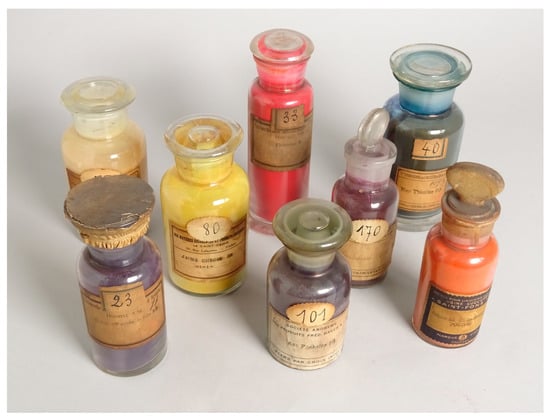This is a detailed photograph of eight vintage glass jars of various sizes and shapes, set against a beige background. The jars, which look old and possibly dusty from long-term storage, are filled with vibrant powders in colors ranging from purple, yellow, red, blue, green, orange, magenta, to peach. Each jar is labeled with a tan, cork-colored tag featuring handwritten numbers: 23, 80, 101, 170, 40, 33, and another barely legible number, possibly 470. The jars have different types of stoppers; most are glass, while two have cork stoppers. The arrangement of the jars showcases their individual character, with noticeable details such as the small orange jar, the medium-sized blue one labeled 40, a tall jar with a red substance, and two purple jars including a tiny one labeled 470. The bottles stand on a flat surface, blending gently into the softly hued background.